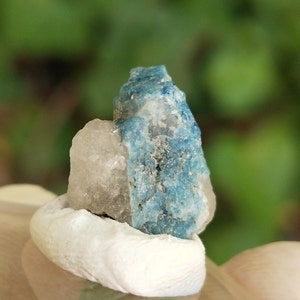The image is a square-shaped, realistic-looking photograph with an out-of-focus green backdrop, suggesting an outdoor setting with trees or foliage. At the center of the photograph lies a striking quartz-like crystal formation consisting of multiple rocks. The tallest rock on the right side is an elongated crystal with a blue hue transitioning to a translucent white, featuring jagged edges and visible cracks. To its left, a white and brown rock rests atop another white rock displaying various shades of white. The background is composed of dark and light green splotches, enhancing the forest-like atmosphere. The rocks appear to be placed or held up carefully, possibly by fingers or on a textured surface. The crystal's intricate structure and the natural blurry backdrop create a harmonious balance in the composition.